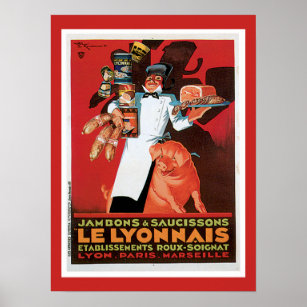This is a vibrant and detailed poster with a retro, cartoonish style. The poster has a primary red background with a white double border, accented by a red outline. It prominently features a cheerful gentleman in a white chef’s coat, black bow tie, and cap, holding an assortment of canned meats and sausages. His right arm is hooked to balance several meats, while his left hand skillfully holds a tray laden with various meats, possibly some Spam. A large shadow of the chef is cast behind him, adding depth to the image. Just below the chef, a friendly, smiling pig stands upright with a blue bow around its right ear, inscribed with yellow letters that read "Jambons et saucissons." The bottom section of the poster includes an ornate brown box with yellow and orange text that states: "Les Lyonnais. Establishments, Rue Soignette. Lyon, Paris, Marseille."